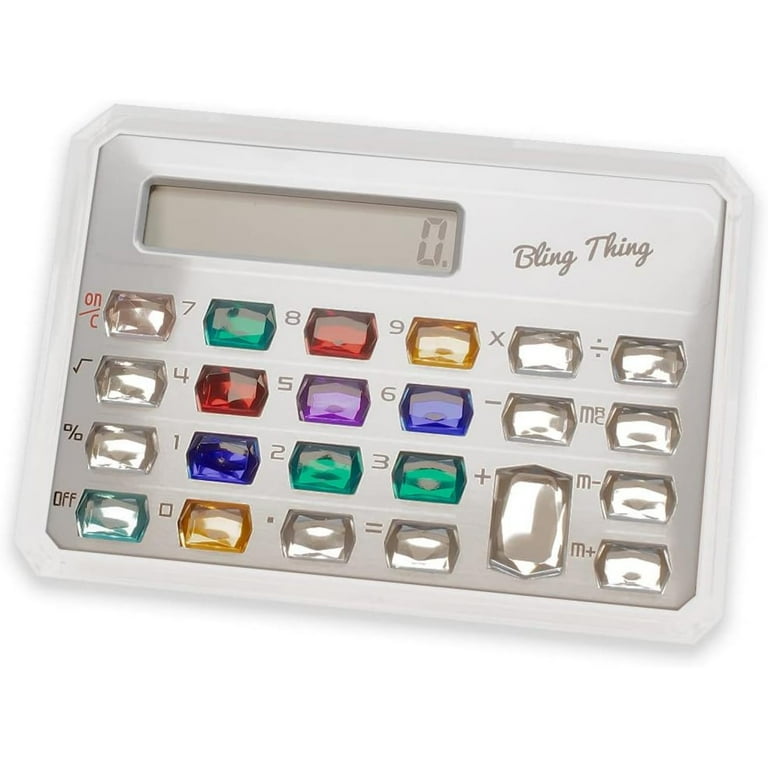This photograph showcases a unique handheld calculator called the "Bling Thing." It features a sleek, rectangular design with beveled edges and a large screen on the top left. The surface is a silvery blue hue, bordered in white, and adorned with an array of colorful, gemstone-like buttons. 

The buttons are arranged in six columns and four rows. Notably, the first three buttons on the top left are diamond-like jewels, followed by a blue button used for 'off'. The number keys are color-coded: yellow for zero and nine, blue for one and six (resembling sapphires), red for four and eight (resembling rubies), and green for two, three, and seven (resembling emeralds). Other operational keys, including plus, memory, multiply, and divide, are also bedazzled with diamond-like colors. 

On the right side, there are two rows of clear gemstones. Towards the middle, colors like blue, orange, brown, purple, red, light blue, and light green add to its vibrant aesthetic. The lettering on the calculator, such as "on" and "A/C" in red, is neatly placed to the left, while the words "Bling Thing" are written prominently on the top right. This extravagant calculator merges functionality with eye-catching elegance.